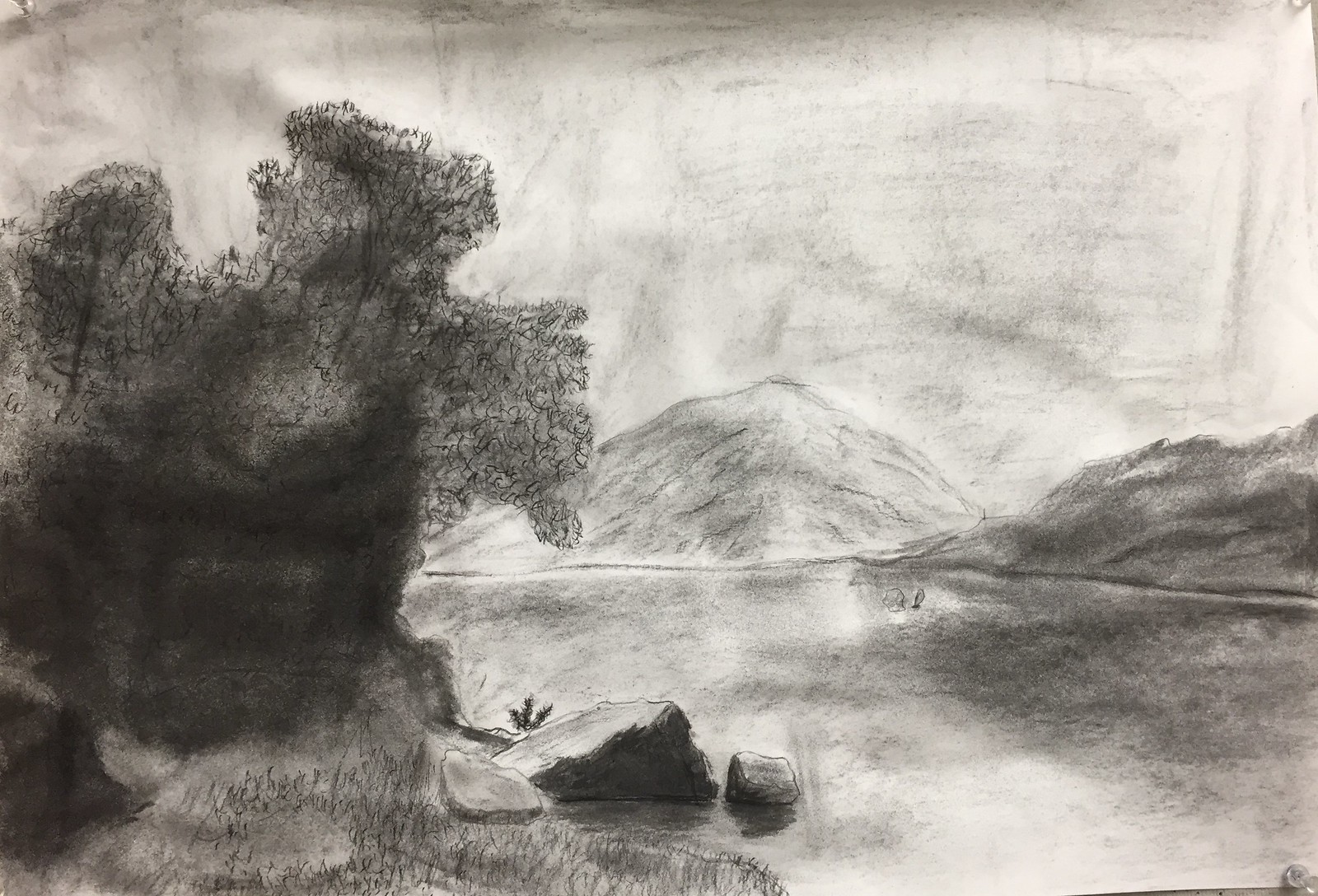This black-and-white landscape sketch captures the serene beauty of a tranquil lake surrounded by nature. In the background, two gentle hills rise, framing the calm waters below. The left side of the sketch features extensive shading, adding depth and contrast to the scene. A prominent, ramp-like rock rests on the shoreline, providing a natural focal point. Adjacent to this rock, on the bottom left, the shoreline emerges clearly, accentuated by a distinctive tree with intricate, web-like patterns in its branches. The tree trunk is enveloped in dark shading, enhancing its prominence in the composition. The sky above is delicately shaded in a lighter tone than the richly detailed foreground, creating a harmonious balance that underscores the black-and-white color scheme.